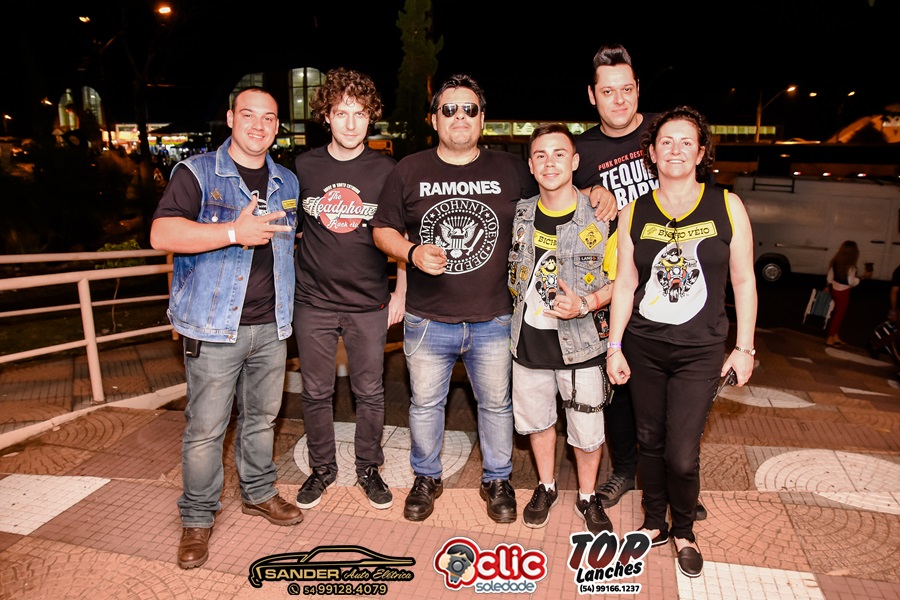In this night-time photograph taken on a patterned tan and rust-colored patio, a group of six Caucasian individuals poses for a picture against a backdrop of illuminated buildings and a dark sky. From left to right, the first person is a man with dark hair, wearing a jean vest over a black t-shirt, blue jeans, and brown shoes, making a gesture with three fingers on his right hand. Next to him is a young man with brown curly hair, dressed in a black t-shirt featuring a red circle with the word "headphone" and brown pants. The center figure is a man with dark hair and black aviator sunglasses, sporting a black "Ramones" t-shirt with white lettering, blue jeans, and black shoes. On his right stands a shorter, younger man, possibly 18 years old, with dark hair. He is clad in a patched jean vest, a black t-shirt with yellow details, blue jean shorts, and black tennis shoes with a leather strap around his left leg. Beside him is a woman wearing a black tank top with a yellow and white graphic design similar to the young man's shirt, paired with black pants and black shoes. Behind her stands a taller man with black hair, wearing a black t-shirt that reads "Tequila Baby."

At the bottom of the image, three logos can be seen, including "Sander" with a number, "Click Soledad," and "Top Launches."